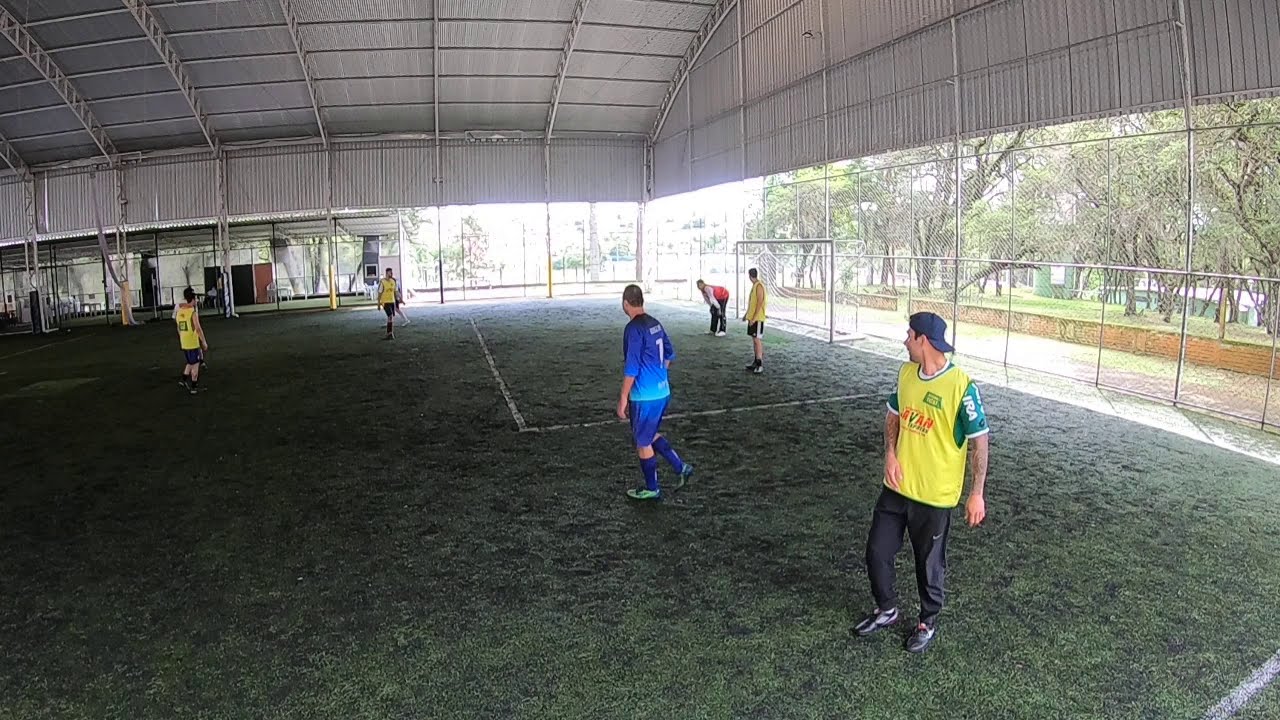The photograph captures a group of men, predominantly between the ages of 20 and 40, playing soccer on a grassy field. This unique field is partially inside a large warehouse-like structure with a sheet metal roof overhead and open sides, providing a semi-outdoor atmosphere in a seemingly tropical environment. There are players in yellow, blue, and green jerseys, some wearing shorts and others in pants, actively engaged in the game: some are running, others walking, and a few observing the action unfold. The field is enclosed with a fence, and there's a goal post visible. The background showcases trees, a road, houses, and distant cityscape, all illuminated by the bright daylight. The canopy's intricate gray railings and patterns are clearly evident above the players. The vivid colors of the scene include blue, yellow, green, brown, beige, gray, and black. One player in a yellow jersey appears in the bottom right corner, another in blue stands center field, and a third player in yellow is situated towards the left background. The setting exudes an energetic sports atmosphere, highlighted by the open-air yet sheltered design of the field.